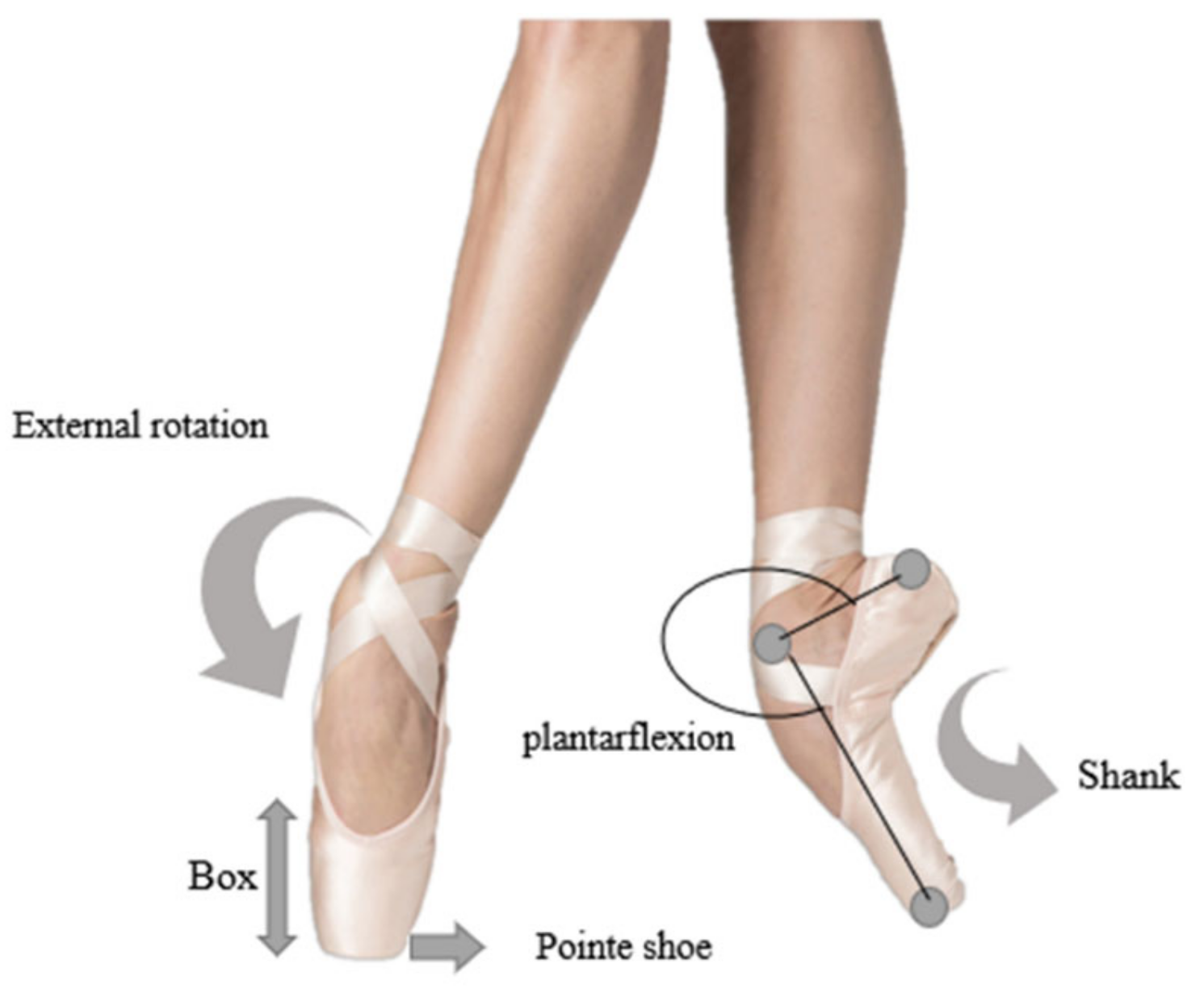The image presents a detailed close-up of a dancer's legs, poised in ballerina shoes against a stark white background. The leg on the left, appearing in a light pink skin tone, extends straight down with a slight leftward curve at the ankle, where the toe is bent. The shoe wraps intricately around the ankle, across the top of the foot, and covers just the top of the toe and sides. The leg on the right bears a shadow near the top and angles slightly to the right before turning inward, showing the top of the foot directly facing left, with its toe bent beneath it. This shoe is marked with gray dots on the heel, ankle, and toe, connected by black lines and a circular line, accompanied by a gray arrow along the arch indicating the "shank."

Text annotations in black decorate the image: "External rotation" is noted at the top left, with a gray arrow depicting rotational movement around the ankle. Below this is the word "box," with a gray line and arrows highlighting the toe area within the shoe. Between the feet, "plantar flexion" is labeled. Another arrow curves along the right foot's arch, labeled "shank," and an arrow on the right points to "point E shoe."

The overall setting, characterized by clear and ample lighting, highlights the elements of posture, structure, and movement, centralizing the dancer's legs and feet in a classical ballet position.